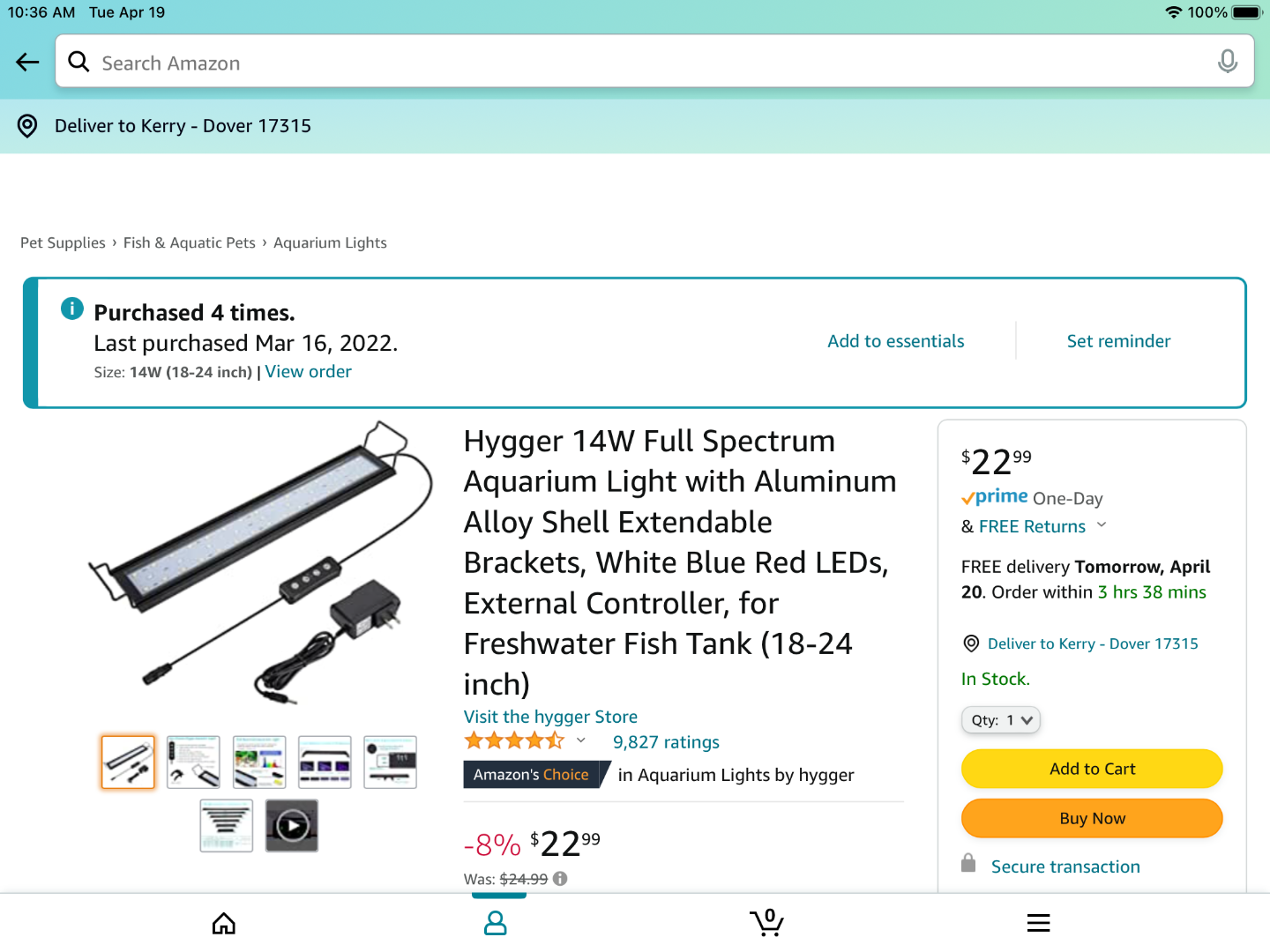This image features a screenshot of an Amazon order placed by Carrie in Dover, with the zip code 17315. The page is viewed on Tuesday, April 19th, at 10:36 AM, with the device showing a 100% battery life and stable connection. The Amazon interface highlights an order under the category of pet supplies, specifically for fish and aquatic pets, focusing on aquarium lights.

The product in question is the HYGGER 14-watt Full Spectrum Aquarium Light, which comes with an aluminum alloy shell and extendable brackets. It boasts white, blue, and red LEDs alongside an external controller suitable for freshwater fish, and fits aquariums measuring 18 to 24 inches. Carrie has purchased this item four times previously, with the last purchase dating back to March 16th, 2022.

The HYGGER store is noted for its high ratings, boasting 9,827 reviews with an approximate rating of 4.25 stars. The product is marked as one of Amazon's choices, signified by a black box with 'Amazon' in white and 'Choice' in orange. The well-illustrated listing includes a comprehensive black-and-white diagram of the aquarium light and its components, five additional images, and a video for further explanation.

Currently, the product is priced at $22.99, reflecting an 8% discount from its original price of $24.99. Prime members benefit from one-day shipping and free returns. The delivery is slated for the following day, April 20th, if the order is placed within the next three hours and 38 minutes. Options to add the item to the cart or buy it immediately are provided, with reminders of a secure transaction displayed in light blue with a lock icon.